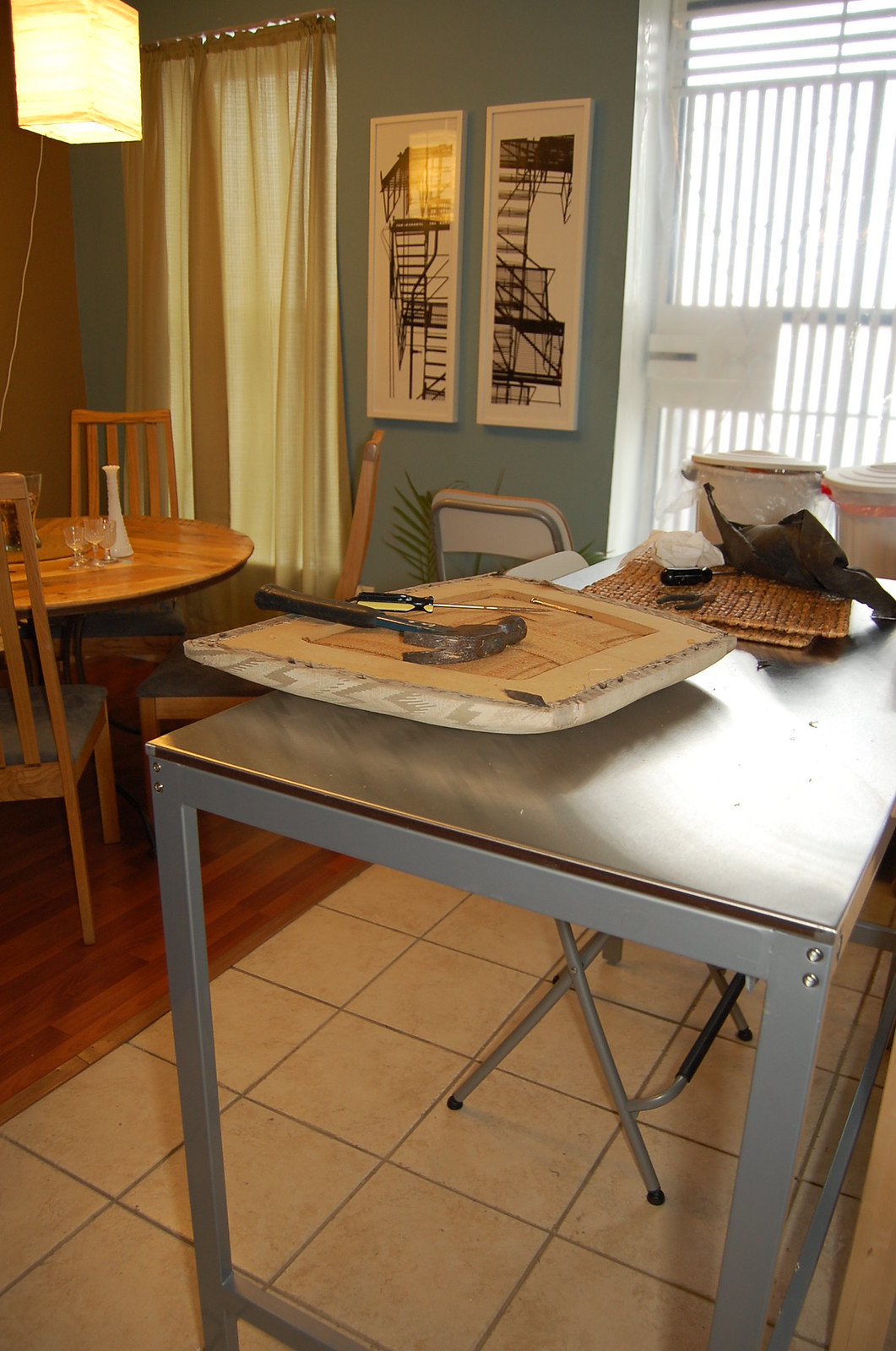The portrait-oriented image captures a cozy scene inside a home. Dominating the central background, a green wall features two vertically oriented, black-and-white framed pictures. To the left, floor-to-ceiling dark curtains add a touch of elegance to the setting. On the right, light streams through a white-grated door, casting a warm glow into the room. A square light fixture in the top left corner further illuminates the space. Below it, a round wooden table, placed on a medium dark-grained wood plank floor, is surrounded by three chairs. The tabletop is adorned with three clear glasses and a tall white flower vase.

In the foreground to the right, a tall table with metal legs and a metal top provides a closer focus. Resting on the table is an upside-down chair cushion, with webbing exposed beneath it. On top of the cushion lies a hammer with its claw facing us, and above it, a black-and-yellow handled screwdriver pointing to the right. Positioned further back on the table are several items, including what appear to be brown woven placemats, a black cloth, and two white canisters, adding to the homely yet functional ambiance of the scene.